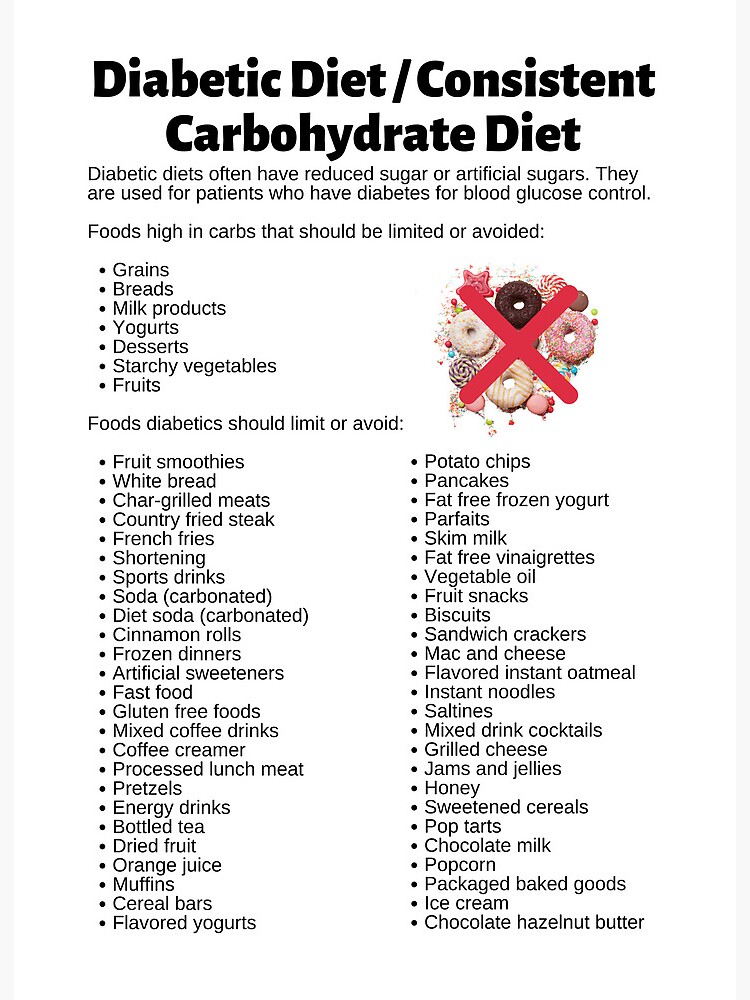This vertical rectangular poster on a white background, printed without any borders, is titled at the top in bold black letters centered: "Diabetic Diet / Consistent Carbohydrate Diet." Below the title, in a normal-sized, left-aligned font, is the explanatory text: "Diabetic diets often have reduced sugar or artificial sugars. They are used for patients who have diabetes for blood glucose control. Foods high in carbs should be limited or avoided." Following this, there are seven bullet points listing: grains, breads, milk products, yogurts, desserts, starchy vegetables, and fruits.

On the right side of this explanatory text, there is a large illustration featuring a big red "X" over images of donuts, candies, and cookies. The next section of text, left-aligned, reads: "Foods diabetics should limit or avoid." This is followed by a long list of specific food items divided into two equal columns containing approximately twenty items each. The list includes foods like fruit smoothies, white bread, char-grilled meats, country fried steak, french fries, artificial sweeteners, diet soda, cinnamon rolls, frozen dinners, fast food, mixed coffee drinks, coffee cream, flavored yogurts, potato chips, energy drinks, orange juice, muffins, flavored instant oatmeal, and more. The comprehensive list is visually detailed with specific mentions of sugary and starchy foods that are not suitable for diabetics.